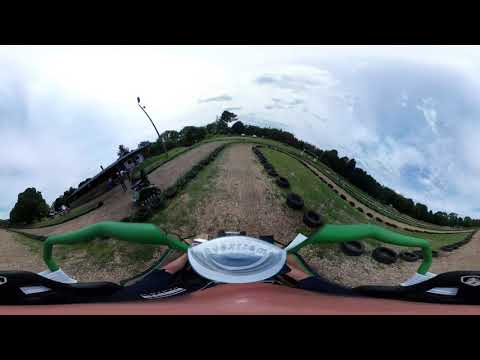This high-definition, GoPro-style photograph, taken from a helmet-mounted camera, captures a scene of a motorcycle — possibly an all-terrain vehicle — on a well-defined dirt path specifically designed for riding. The image is bordered by black rectangular shapes at the top and bottom, adding to the widescreen format.

The rider's perspective showcases the two handlebars, with their arms presumably below them, and a blurred silver object, likely the speedometer, at the center. The dirt path, lined with stacked tires on both sides, winds its way up a steep incline towards a peak before curving to the right and descending. This pathway is bounded by hedges and grassy areas, with additional dirt tracks adjacent on either side.

Above the trail, a partly cloudy sky adds a soft light to the scene, further highlighting the curving, undulating terrain lined with trees on both sides. The vegetation and tires guide the eye along the track, suggesting a circular route that dips and rises, providing an adventurous and scenic ride. The overall atmosphere is one of a mildly cloudy yet dry day, perfect for an exhilarating off-road experience.